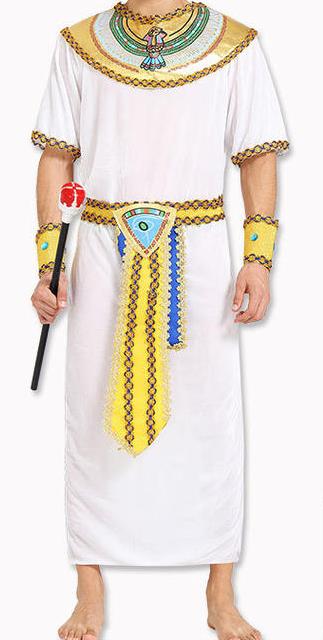The image showcases a model dressed in an elaborate Egyptian-themed costume, depicted from the neck down to the feet, accentuating the intricate details of the outfit. The model wears a long, white garment resembling a robe or a dress, with short sleeves. The clothing features a striking yellow and golden belt adorned with Egyptian symbols, resembling a shield-like belt buckle. Extending vertically from the buckle is a yellow sash that reaches past the knees. Around the neck, there's a substantial collar that spans from shoulder to shoulder, embellished with what appears to be Egyptian iconography and a green bird motif.

Golden wrist gauntlets, rather than full gloves, adorn the model’s arms, emphasizing the outfit's regal essence. In the model's right hand is a scepter—a black rod capped with a red gem or jewel, which some describe as resembling a small crown with a velvet top. The model's bare feet are visible, further contributing to the traditional and historical ambiance of the ensemble. The overall impression is that of an Egyptian prince or deity, with thoughtfully placed accessories and symbols enhancing the authenticity of the portrayal.